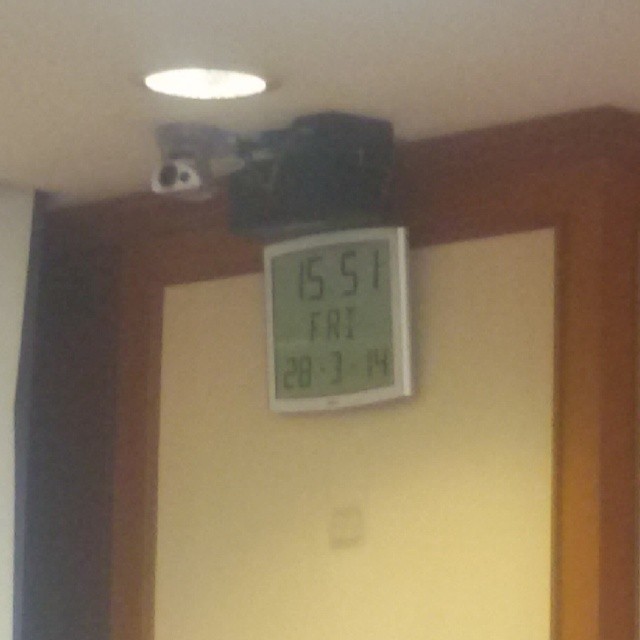This slightly grainy photograph captures a ceiling-mounted projector with a sleek silver and black design. Directly above the projector, a soft white light casts a gentle glow, illuminating the scene. Beneath the projector, a white wood trim with an orangey hue adds a touch of warmth to the setting. On a white portion of the wall below the trim, a silver-mounted digital display prominently shows the date and time—1551, Friday 28-3-14—in clear black font. Faintly in the lower part of the image, a subtle black object is discernible against the wall, contributing to the photograph's textured, somewhat fuzzy appearance while still retaining enough clarity to distinguish key elements.